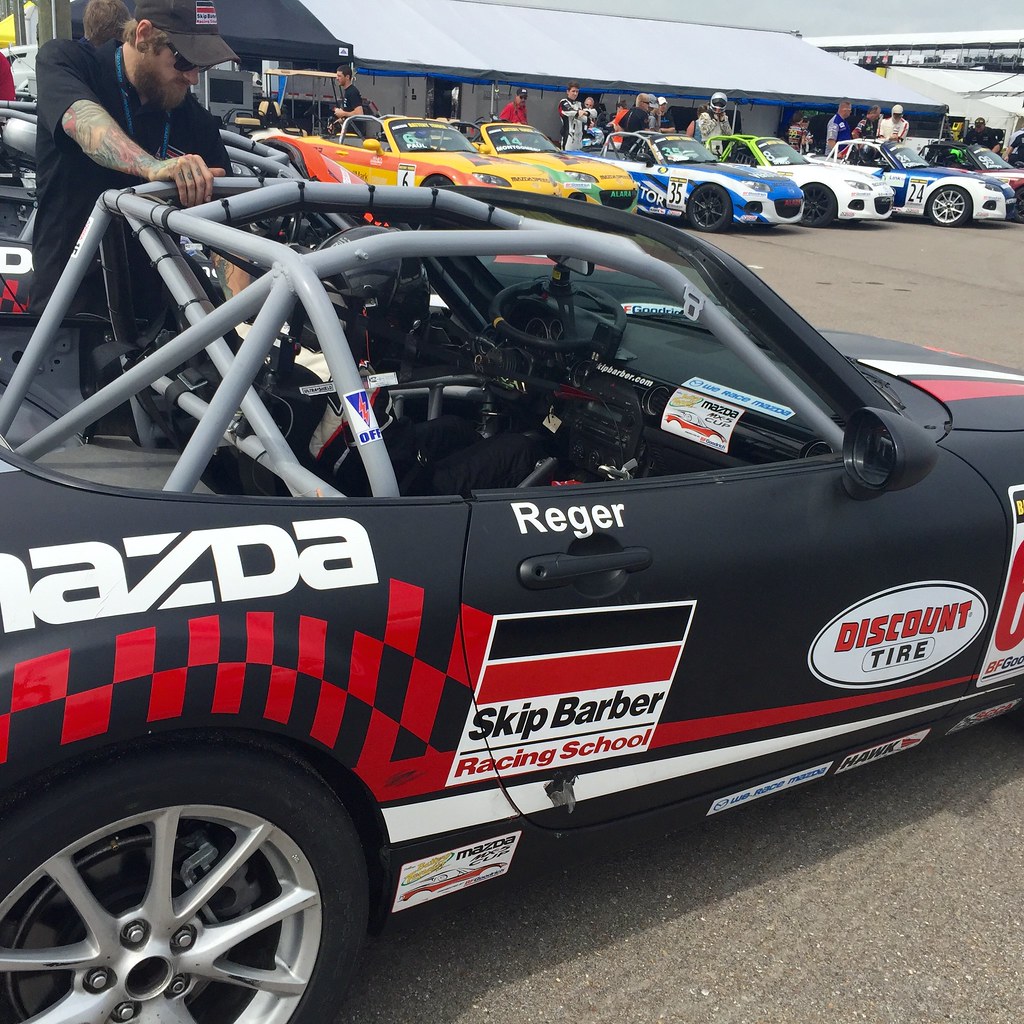The image captures a scene at a racetrack featuring a black Mazda Miata race car prominently adorned with advertisements. The race car, which has a flat black paint job and red checker patterns on the sides, showcases various sponsors including Discount Tire and Skip Barber Racing School. The name "Rieger" is displayed in white text on the passenger side door. A white square with black and red stripes features the Skip Barber Racing School logo, while a white oval highlights the Discount Tire logo. The car is equipped with a light gray roll cage, and the driver, dressed in an all-black racing suit and helmet, is visible inside.

In the foreground, a man in a black short-sleeved shirt, black hat, and sunglasses, with a full-sleeve tattoo on one arm and a blue lanyard, leans on the car, discussing preparations with the driver. Nearby, a technician in a black polo shirt carefully inspects the car's wheels and engine, ensuring everything is functioning properly. Behind this scene, a row of similarly modified and branded Miata race cars are lined up, surrounded by pit crews and drivers, indicating a race is about to begin. The atmosphere is charged with anticipation as teams make last-minute adjustments to their vehicles.